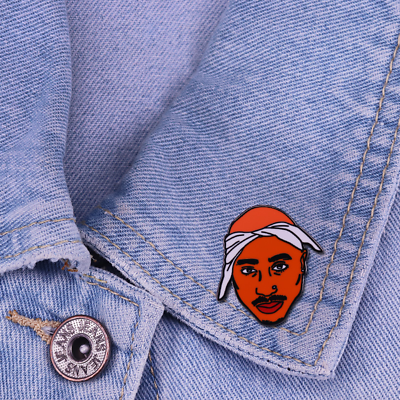The image is a close-up of a light blue denim jacket, showcasing a circular button at the top that reads "JEANS" around its edge. Prominently featured on the left lapel is a detailed pin of the iconic rapper Tupac Shakur. The pin is designed with a light brown base, displaying Tupac's facial features, including his eyes, eyebrows, nose, a slight mustache, and his lips. His head is adorned with his trademark white bandana tied around it. The denim material and button suggest a classic, simple jacket style, with the unique and striking Tupac pin adding a personal touch. The composition is tightly cropped, focusing primarily on the pin and the button, with most of the denim fabric occupying the background.